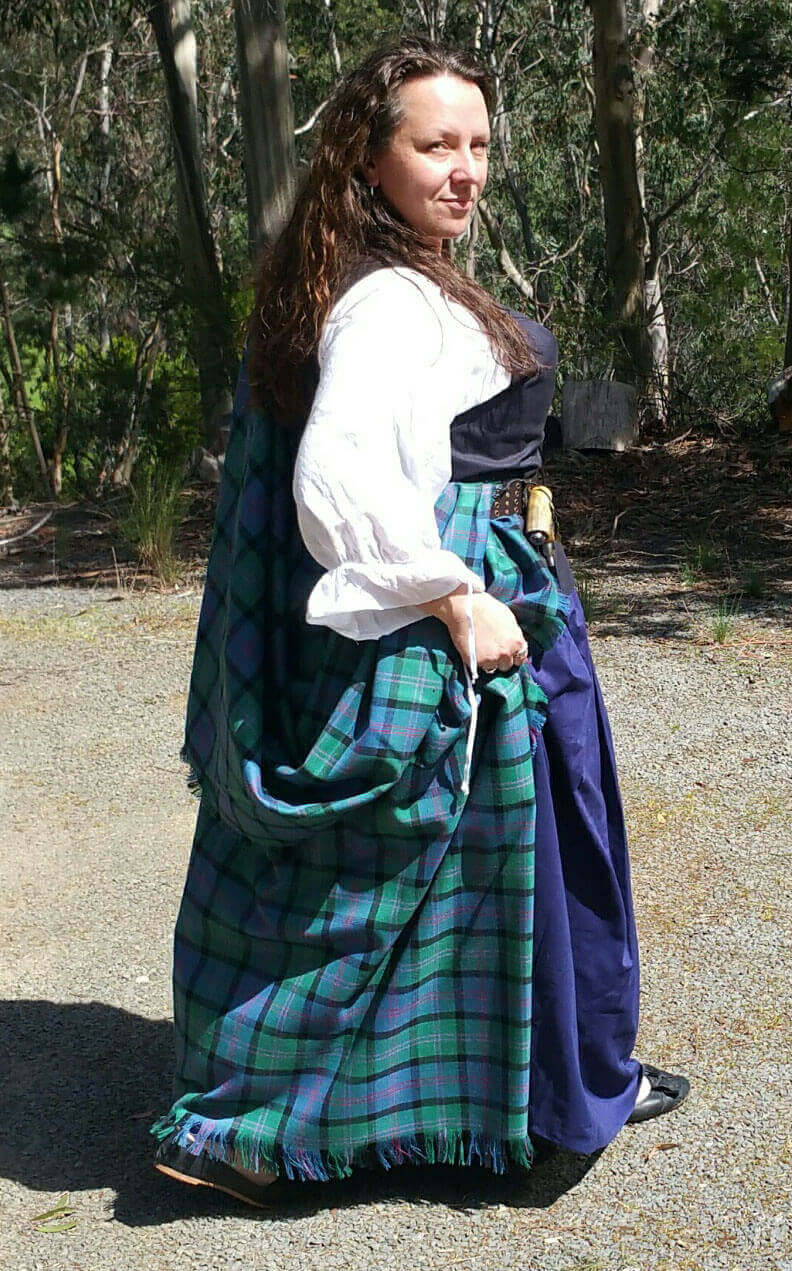The image features a woman, dressed in medieval-inspired attire, standing on a dry, grayish ground that has scattered brown spots. Her detailed outfit includes a white, long-sleeved, puffy blouse with ruffled cuffs, over which she wears a dark, form-fitting bodice. The blouse and bodice ensemble extends into a dark blue skirt that reaches her feet. Draped over her shoulder and waist, she has a shawl featuring a checkered pattern with shades of light blue, green, and a hint of purple, with frayed ends. Her dark brown, wavy hair cascades down to the middle of her back, with some strands draped over her shoulder. She is standing in a side profile facing right, with her head slightly turned towards the camera, revealing a bit of her face. Her footwear includes small black shoes, with a glimpse of her skin at the top. The background is a dense forest composed of a thick array of green trees, stretching out as far as the eye can see. The overall scene suggests she might be at a historical reenactment event or a medieval fair.